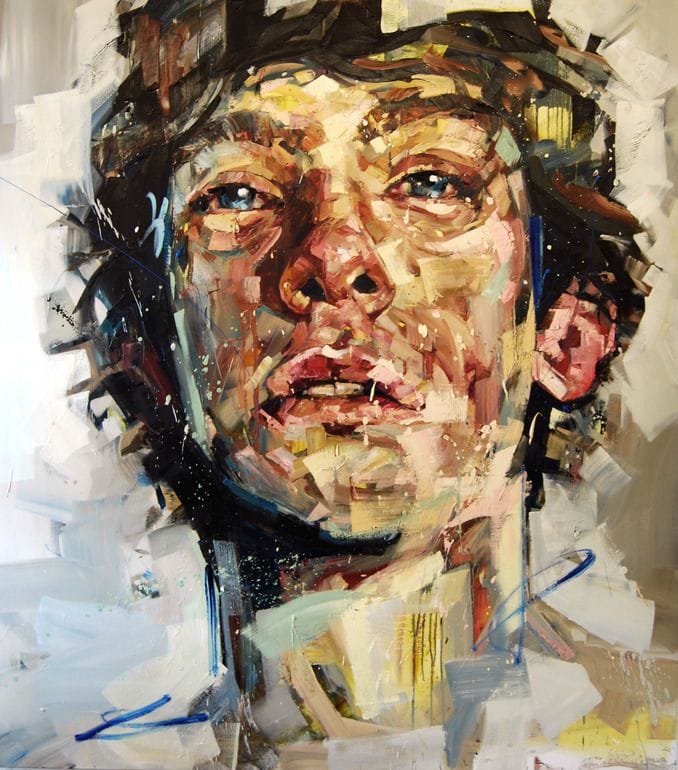The image is a vibrant, abstract painting of a man's face and neck, created using a mix of oil, canvas, and watercolor techniques. The man has short, somewhat curly brown hair, with some strands covering his ears, and striking blue eyes. His expression is nuanced, with his mouth slightly open, revealing his front teeth, lending him a somber appearance as if he might be crying. The artist employed a diverse palette, incorporating reds, browns, yellows, and blues to form a patchwork effect across both his face and neck. Various colored streaks, including red and yellow, are prominent on his face, while blue hues are noticeable below his chin. The background of the painting is composed of mostly neutral colors, also applied in a patchwork style, framing the man's face and enhancing the emotional depth of the portrait.